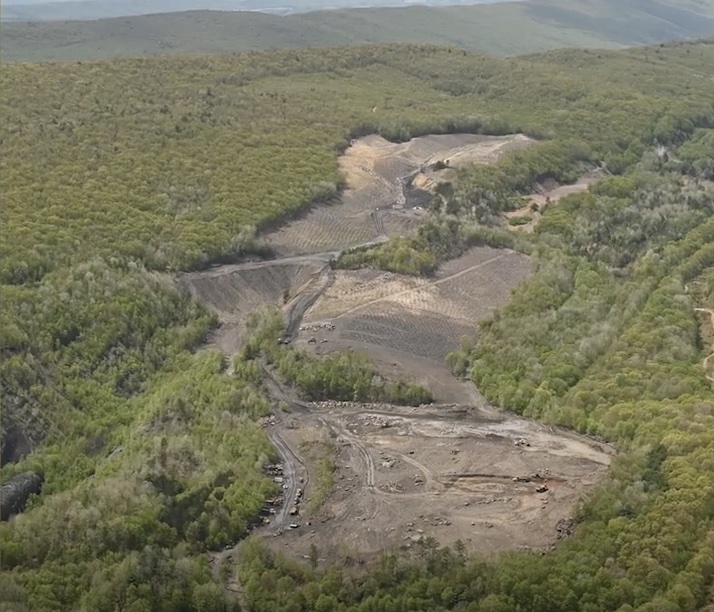The photograph is an aerial view capturing a broad, rural landscape dominated by a dense forest and hilly terrain, with more pronounced mountainous features in the distance. In the center of the image, there is a large, conspicuous clearing where the trees have been completely removed, revealing a vast expanse of dirt and smaller rocks. This cleared area covers about two-thirds of the height and a third of the width of the photograph. Scattered throughout this barren section are construction vehicles and logging trucks, indicating active logging operations. Visible lines and stumps mark the paths where trees have been cut down. A road snakes into the clearing from the right side, further emphasizing the human activity amidst the natural landscape. The mountains in the background have peaks that are nearly flat, contrasting with the rugged, forested hills surrounding the cleared zone.